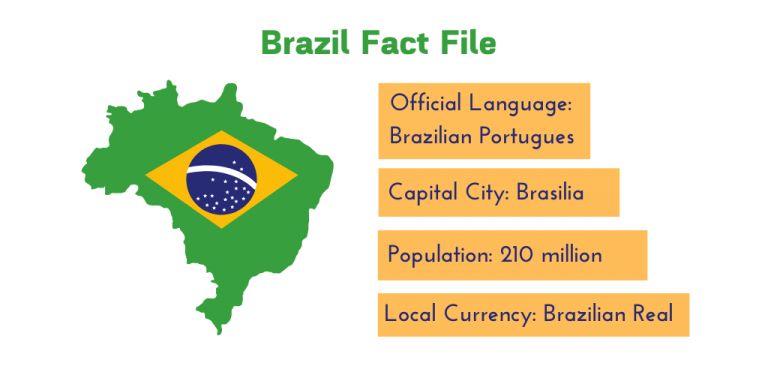The infographic titled "Brazil Fact File" provides a concise overview of key information about Brazil, presented with a clean and colorful design that mirrors the national flag. 

At the forefront, on a white background, is a green outline map of Brazil. This map is superimposed onto a large, horizontally oriented yellow diamond that stretches side-to-side. Centered within the diamond is a blue circle featuring a white horizontal stripe adorned with small white stars, reflecting the central emblem found on the Brazilian flag.

The title "Brazil Fact File" is situated prominently in the same green as the map. Below the title, the infographic is divided into several yellow boxes, each containing text in blue to match the flag's color scheme. These boxes succinctly list pertinent details about the country:

- **Official Language:** Brazilian Portuguese
- **Capital City:** Brasília
- **Population:** 210 million
- **Local Currency:** Brazilian Real

Overall, the design is minimalistic yet effective, focusing on a quick delivery of basic facts without unnecessary embellishments.